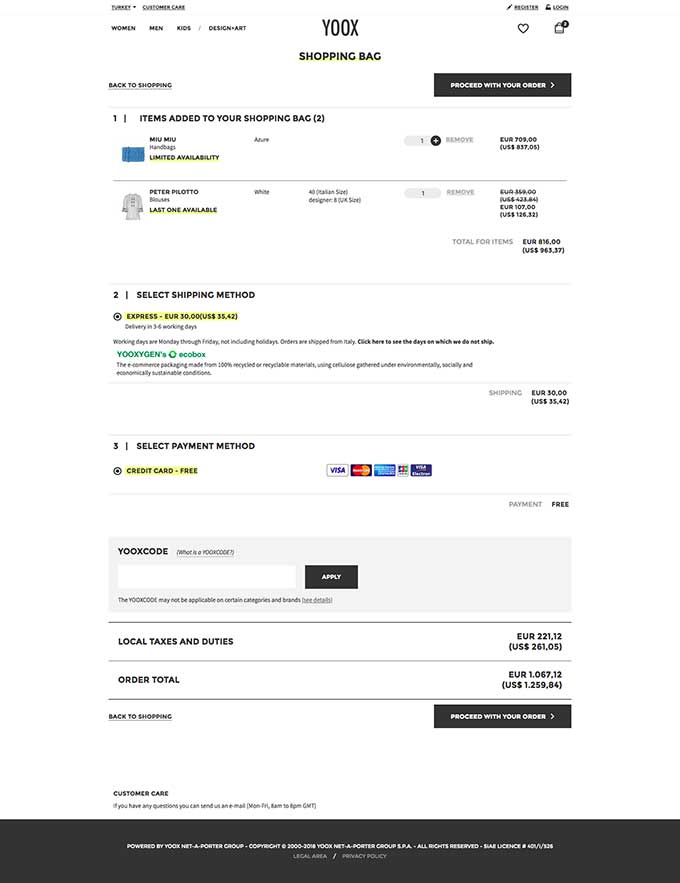Here is a detailed and cleaned-up description for the given image:

"Displayed on the screen is the shopping bag page of the YOOX website. The interface is clean, predominantly white with crisp black text. The shopping cart contains two items, specifically a t-shirt and a handbag, though the details are not entirely legible. The checkout process is outlined in clear steps: 'Step 1: Review items', 'Step 2: Select shipping method', and 'Step 3: Select payment method.' Various payment options are visible, including Visa, MasterCard, American Express, and Discover logos. There is also a section to apply a promo code, along with a breakdown of local taxes and duties. The order total is displayed but the exact numbers are not clearly readable. At the bottom of the page, a black bar prominently features the option to 'Proceed with your order.' The overall design is minimalist and user-friendly, with a black footer completing the webpage’s aesthetic."